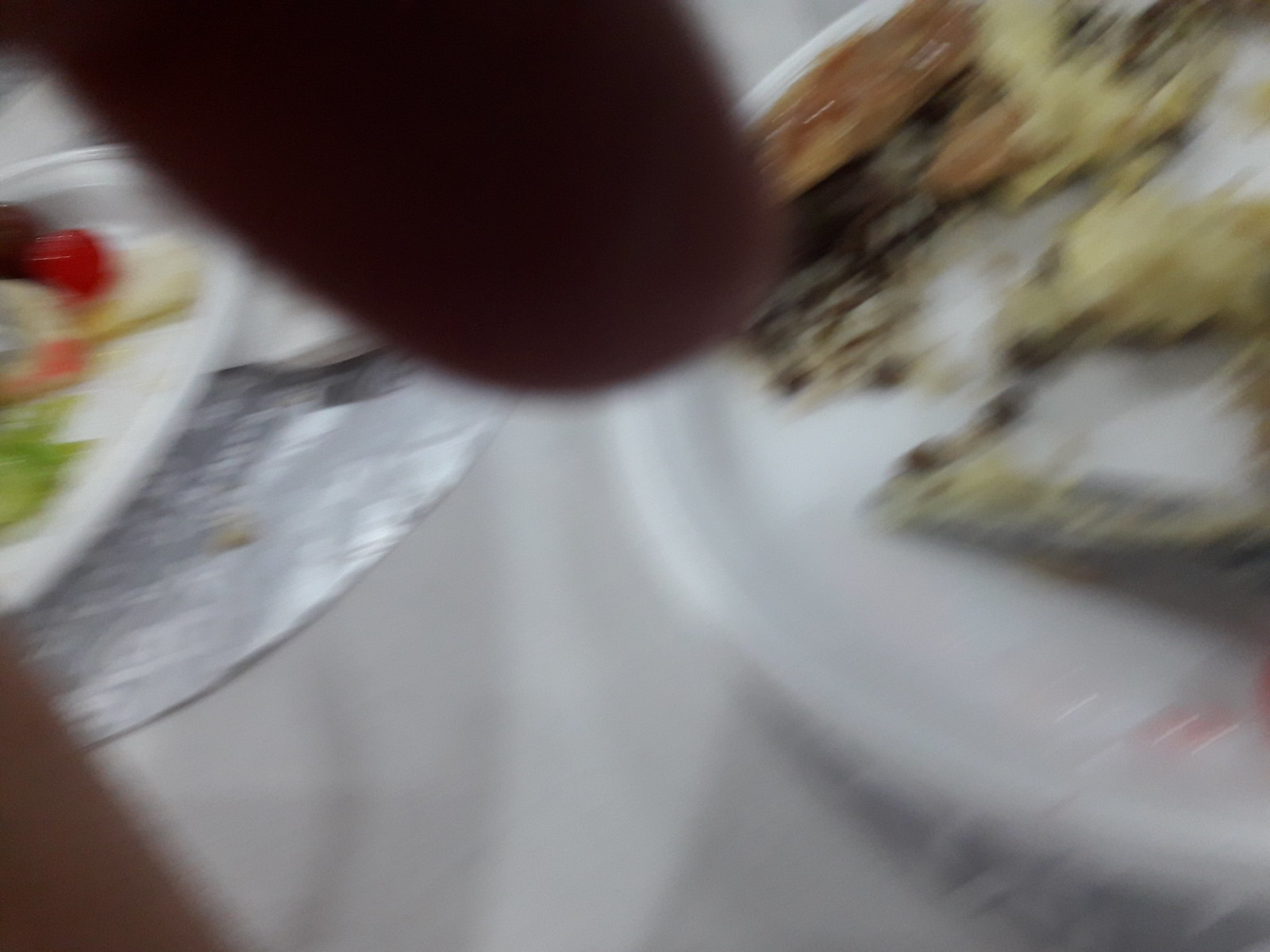This is a color photograph that is very blurry, showing part of a person’s finger, along with a glimpse of their hand and arm, overshadowing two plates of food on a table. In the upper left corner, a dark brown object, likely the person's finger, protrudes into the frame, with another part of the hand seen in the lower left corner. The table is covered with a crumpled, greyish tablecloth.

On the left side of the image, there is a partially visible silver plate with white writing. Placed on top of this silver plate is a smaller, oval-shaped plate, featuring what appears to be a variety of food items, including red berries and green vegetables. A silver spoon is just visible, extending from the edge of the smaller plate.

To the right, occupying about half of the photo, is a larger, round white plate. There is a small red logo towards the bottom edge, partially obscured by what seems to be crumpled plastic wrap. The food on this plate appears to include a slice of a brown and yellow cake, possibly fruitcake, scattered with black spots. Additionally, there seems to be a clump of white food and a crusted piece filled with green, drizzled with some sauce on the same plate. The image captures only parts of these elements due to the blurriness and partial obstructions.